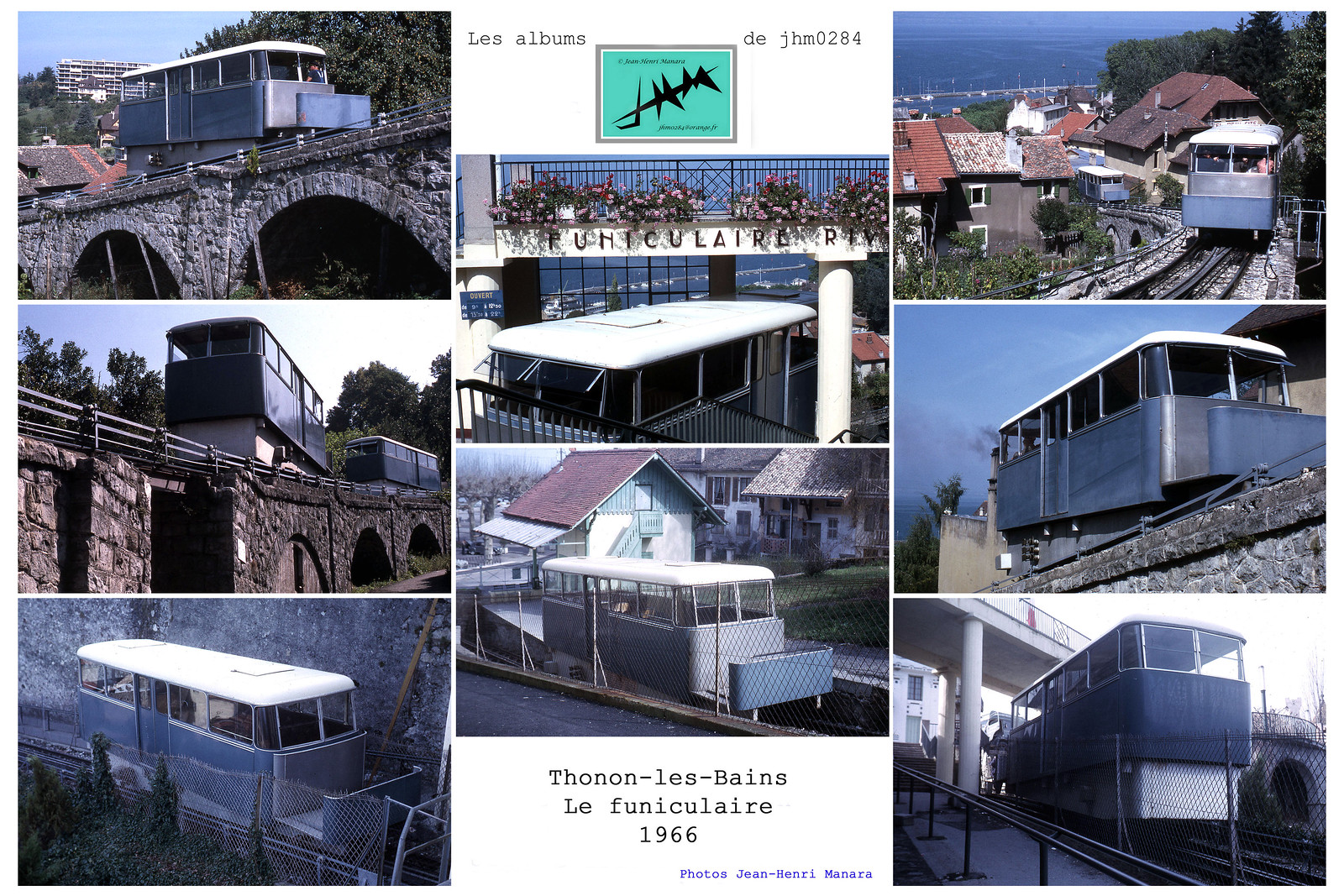The image is a brochure cover featuring a collage of eight vertically arranged photographs that showcase a distinctive blue tram service from various perspectives. On the left side, three images depict the blue and white trams traveling on tracks over stone bridges, with scenic backdrops of trees, buildings, and water bodies. The central column of two photos includes a top image of a building adorned with flowers and labeled "Funiculaire Riv," featuring large white pillars and trams stationed nearby, with a view of ships on the water in the background. The bottom central photo shows the tram moving along its tracks with houses in the distance. On the right side, three vertically aligned images capture the trams from different angles, highlighting their transit over scenic routes with bridges and waterfront vistas. The brochure prominently features a logo at the top center with a turquoise background, outlined in grey and white, containing a stylized "JHM" and the text "Corporate Jean-Henri Manara" along with "J H M 0284." The text "Les Albums" appears on the left side, while "DHM 0284" is on the right side. The bottom of the image includes the text "Thonin-Les-Bains," "Le Funiculaire 1966," and "Photos Jean-Henri Manara." The tram's distinctive livery, with its steel blue body and white roof, is consistent across all images, projecting the vintage charm of this historic public transport.